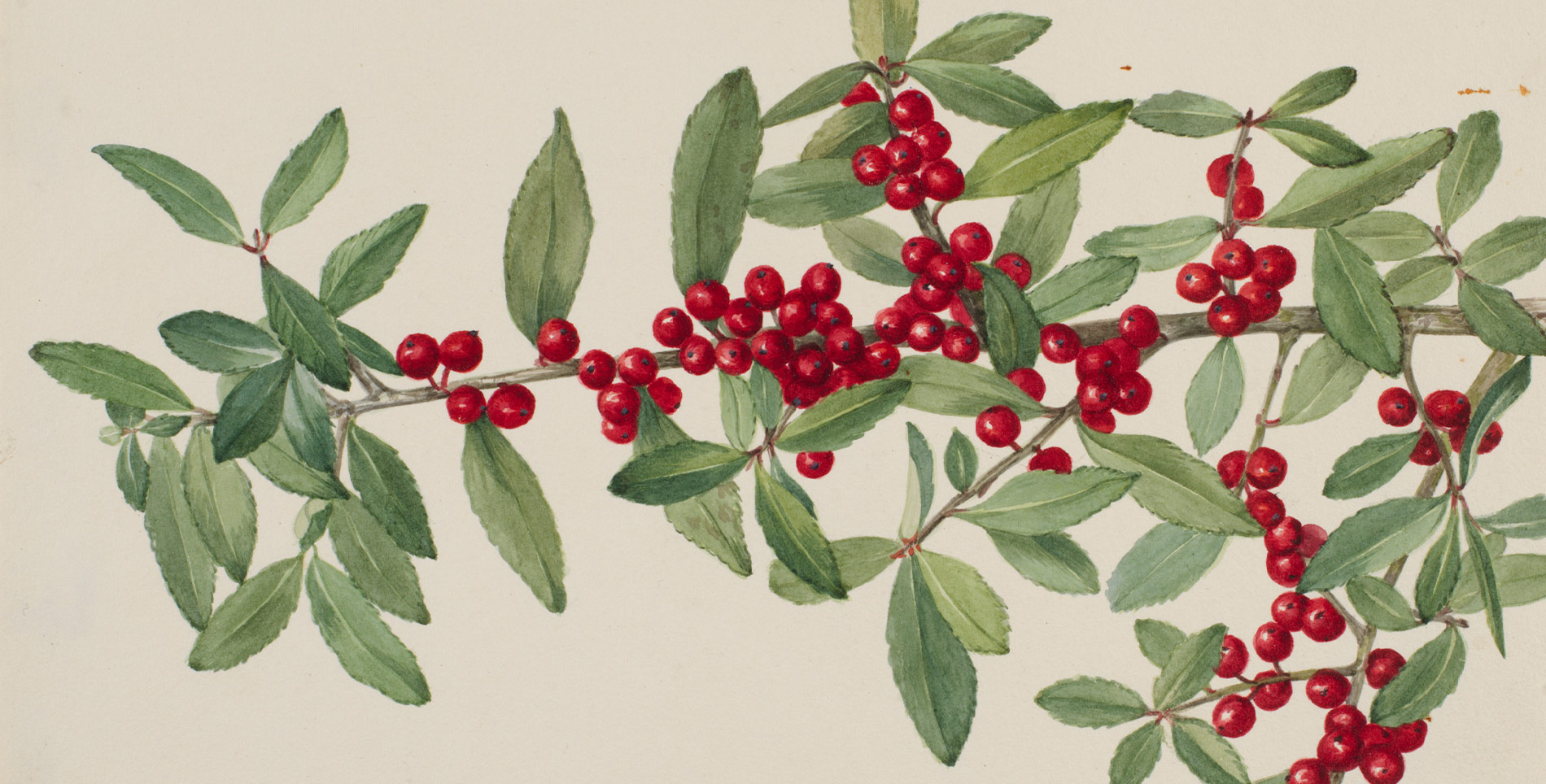The image is a detailed illustration reminiscent of a Victorian sketch from a natural history book. It depicts a large tree or bush branch extending from the right side almost to the left side of the landscape-oriented print, set against an off-white or light tan background that resembles aged paper. The branch is adorned with smaller sub-branches sprouting both upward and downward, each bearing numerous oval to diamond-shaped dark green leaves. Interspersed among these leaves are abundant small, circular red berries. Overall, the artwork features dozens of green leaves and about a hundred red berries, giving it a lush, vibrant appearance.